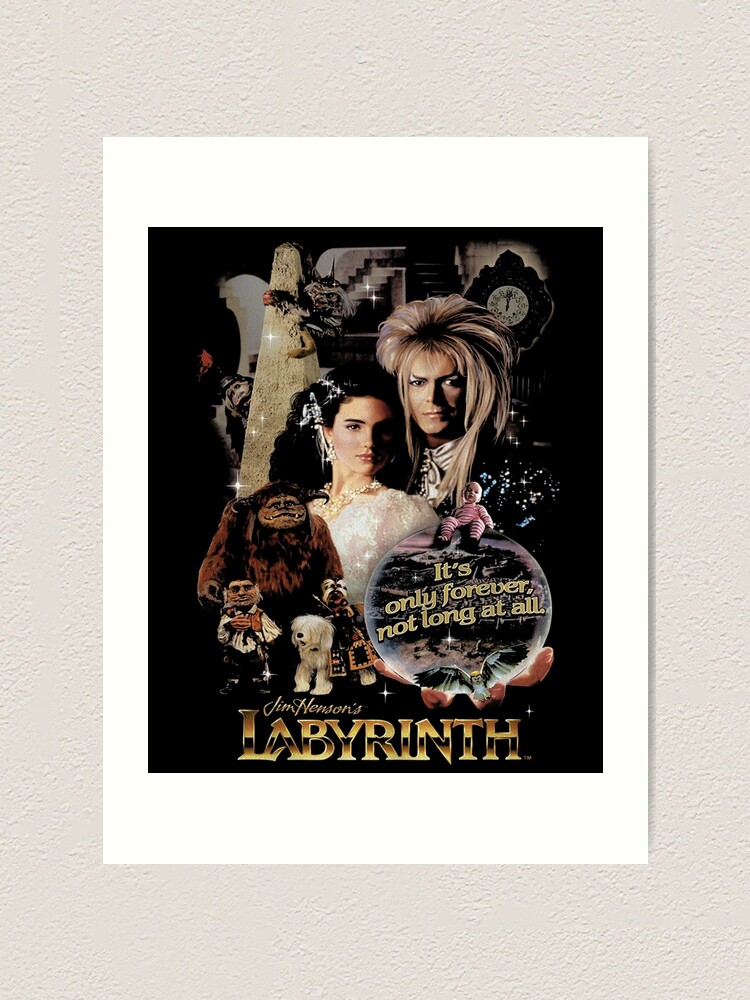This framed movie poster for "Labyrinth" features a striking black background with a white and gray mat. Central to the poster is an assortment of characters and text that pop vividly against the dark backdrop. The prominent figure is a Caucasian man, decorated in flamboyant 1980s style, with long blonde hair that cascades to his right side, reminiscent of David Bowie's iconic look. He is holding a yellow text bubble that reads "It's only forever, not long at all." Standing in front of him is a young girl donned in a pristine white dress and upkept dark hair. Surrounding them are various mythological and fantastical creatures, including a gorilla-like being, a horned monster, small gargoyles, and a baby in red and white striped clothing perched on a small bulb. In the hazy background, a clock and other indistinct objects add to the mystical ambiance. At the bottom, the title "Jim Henson's Labyrinth" is elegantly displayed in large metallic gold letters. The entire poster radiates a nostalgic, whimsical energy, encapsulated within the speckled gray matting that frames it.